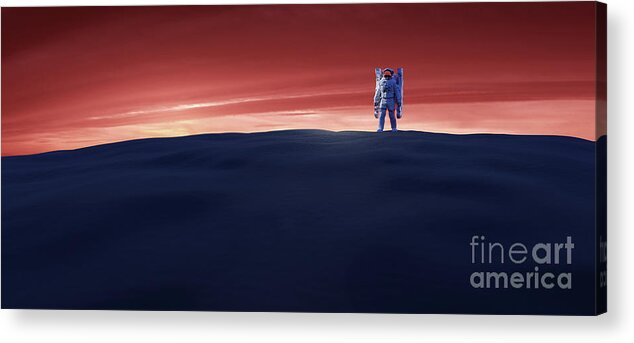This is a detailed depiction of a canvas painting, appearing slightly three-dimensional due to a faint border and a drop shadow on the right side. Dominating the scene is an astronaut in a white space suit with a reddish visor, standing on a gray, barren, and slightly sloped moon-like landscape. The sky above creates a dramatic backdrop, transitioning from a darker orange and brick-red at the top left and right to a lighter pinkish hue, with an ethereal, sun-like glow emerging in the center-left amidst pink and red clouds, giving the feeling of a surreal alien sunset. The lower right-hand corner of the painting features the text "Fine Art America" in lowercase gray letters.